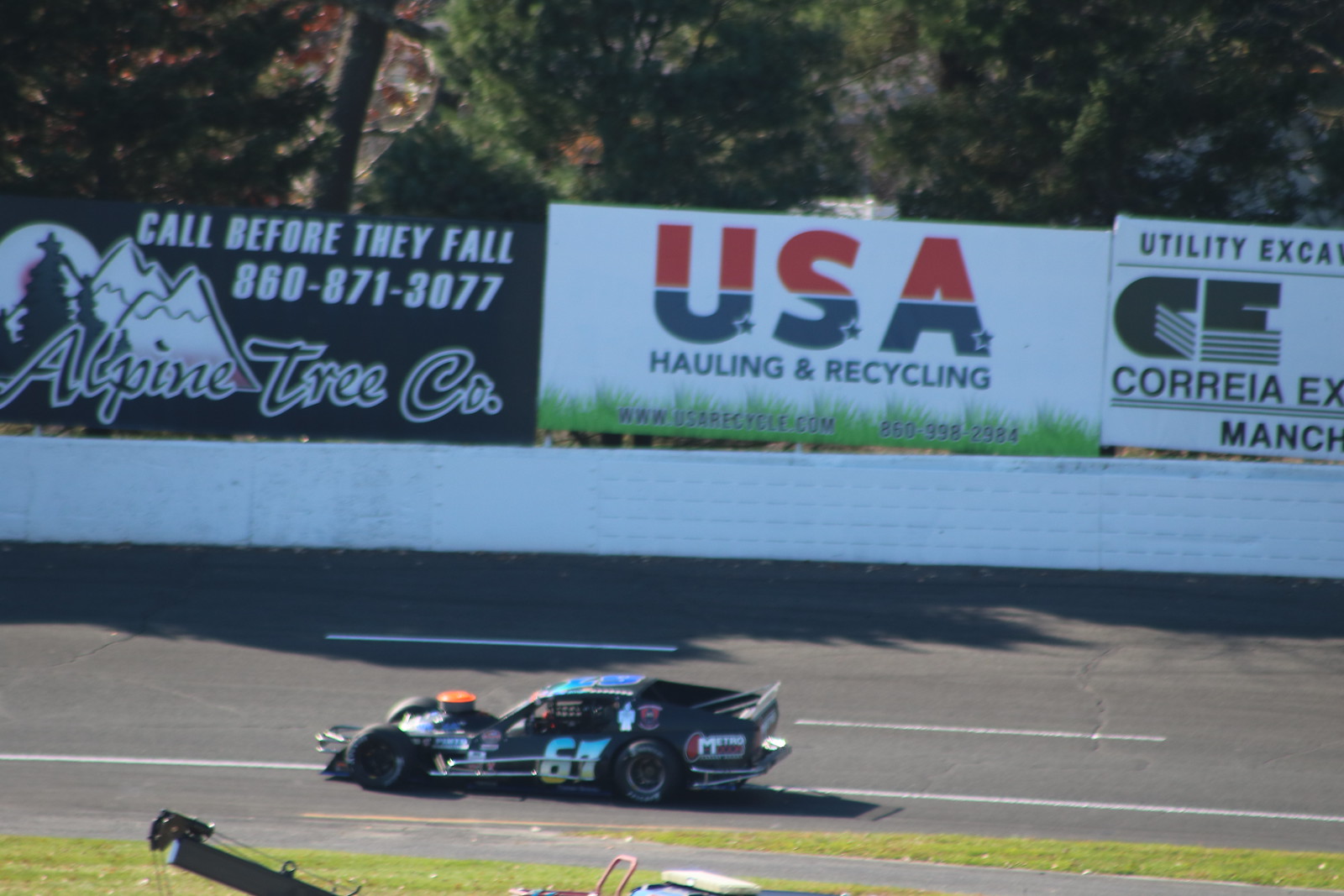The image features a sleek race car, primarily black with a teal-colored roof fading to white at the bottom, speeding down the track. Displayed prominently on its side is the number 67, along with various sponsor logos in small text, including Metro. The car's low profile and visible front engine suggest a design reminiscent of both F1 and traditional sports cars. Surrounding the track is a grassy field, where a piece of machinery, possibly a crane, is visible. In the background, beyond a white wall, numerous billboards advertise sponsorships such as USA Hauling and Recycling, "Call Before They Fall" Alpine Tree Company with their contact number 860-871-3077, and what appears to be Corea Utility Excavator. Towering trees hover over the billboards, adding a natural contrast to the vivid racing scene.